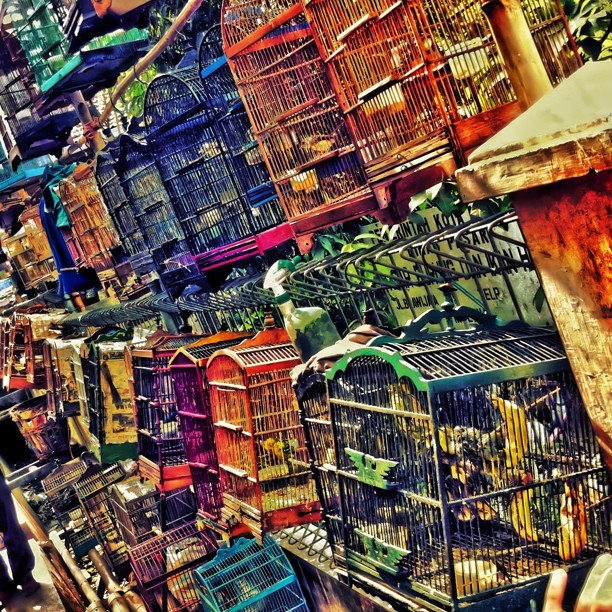This photograph showcases a vibrant array of bird cages, potentially in a bustling pet or bird store. The cages, constructed with black metal railings, are adorned in an array of striking colors, including red, yellow, orange, green, blue, purple, dark green, cyan, and violet. Each cage, square in shape with an arched top, is either stacked on tables or suspended from hooks, creating a visually dynamic scene. The cages feature various symbols on the front, adding to their intricate design. Among the cages, a person's outline is visible, wearing black pants and shoes. Additionally, spray bottles, possibly for water, are scattered around. The photograph provides a sense of an outdoor setting, as illustrated by the concrete bollard to the right and the subtle hint of a road behind, giving the impression that the rows of bird cages, vertically stacked and slightly set back at each level, are being viewed in a market-like environment. Although birds are likely in the cages, they are not clearly visible.